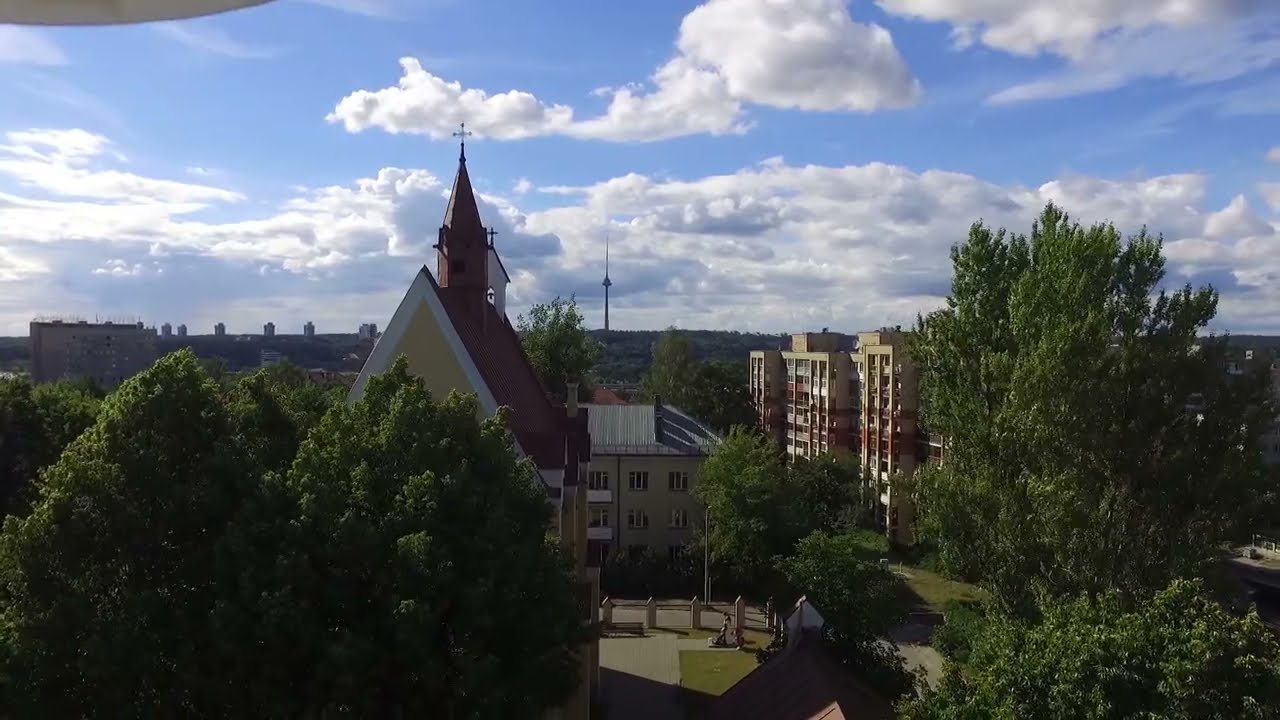This drone-captured color photograph, taken from above and in landscape orientation, showcases a small town on a clear day. Central to the image, though slightly off-center to the left, stands a church with a steep A-line roof and a spire topped by a cross. The church is partially obscured by dense green trees in the foreground. To the right of the church are several multi-story buildings with a beige stucco finish, and smaller buildings can be seen further in the distance. The bottom foreground features a parking area with a beige paved surface and a fence. The right side of the image has even more buildings set amongst a scattering of trees, including taller structures that seem to reach 10 to 15 stories high. The horizon shows a mix of trees and buildings beneath a vast blue sky dotted with poofy white clouds.